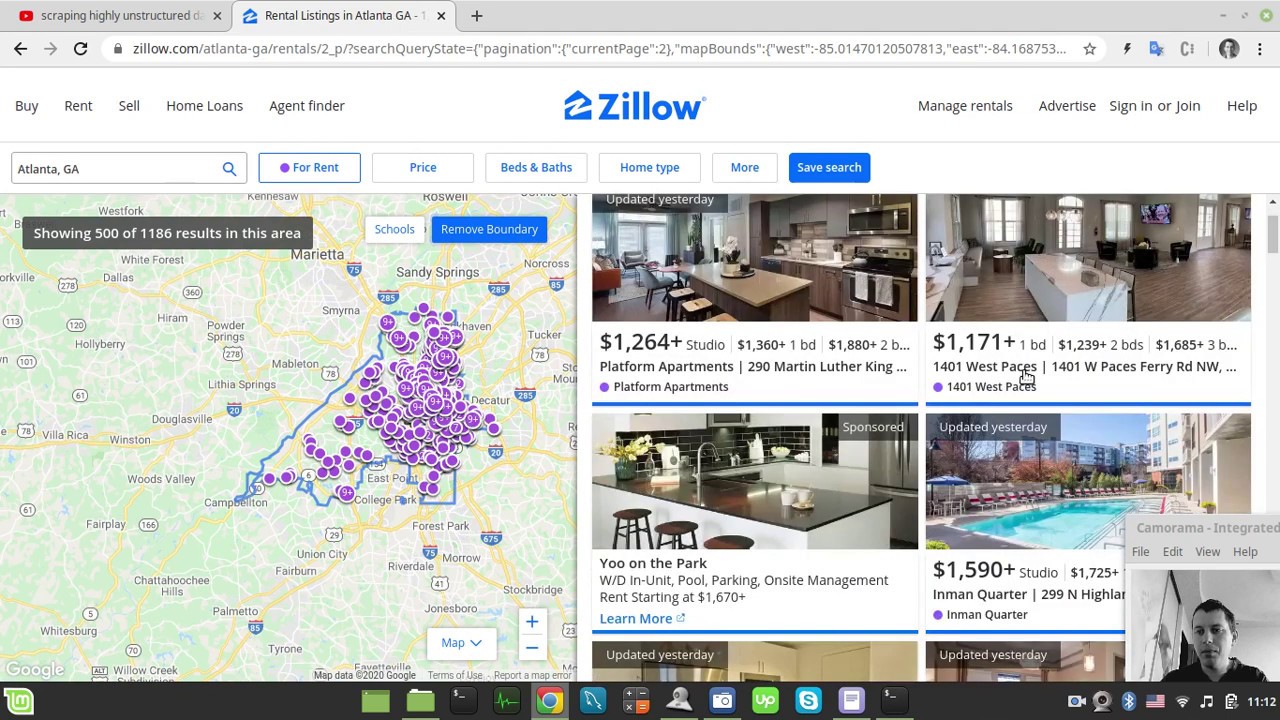A detailed screenshot of a computer screen showcases two browser tabs. One tab is titled "scraping highly unstructured," while the active tab displays "rental listings in Atlanta, Georgia" on Zillow's website. Centered at the top of the screen, the Zillow logo in blue appears within a white navigation bar.

On the navigation bar's left side, the tabs "Buy," "Rent," "Sell," "Home Loans," and "Agent Finder" are visible. To the right of the Zillow logo, options include "Manage Rentals," "Advertise," followed by a gray "Sign in" or "Join," and "Help."

Below the navigation bar, a detailed map of Atlanta, Georgia occupies the screen, featuring various real estate search options like "For Rent," "Price," "Beds & Baths," "Home Type," "More," and "Save Search," with "Save Search" highlighted in blue. The selected "For Rent" option displays a regional map, extending to places like Marietta, Georgia, and shows 500 out of 1,186 available rental listings. An option to "Remove Boundary" is also accessible.

On the right side of the interface, four property images provide a preview of the listings, including price ranges from $1,171 to $1,590 for relatively small rental units. An avatar or a picture of the user browsing the listings might be present, possibly indicating a customer support interaction in progress.